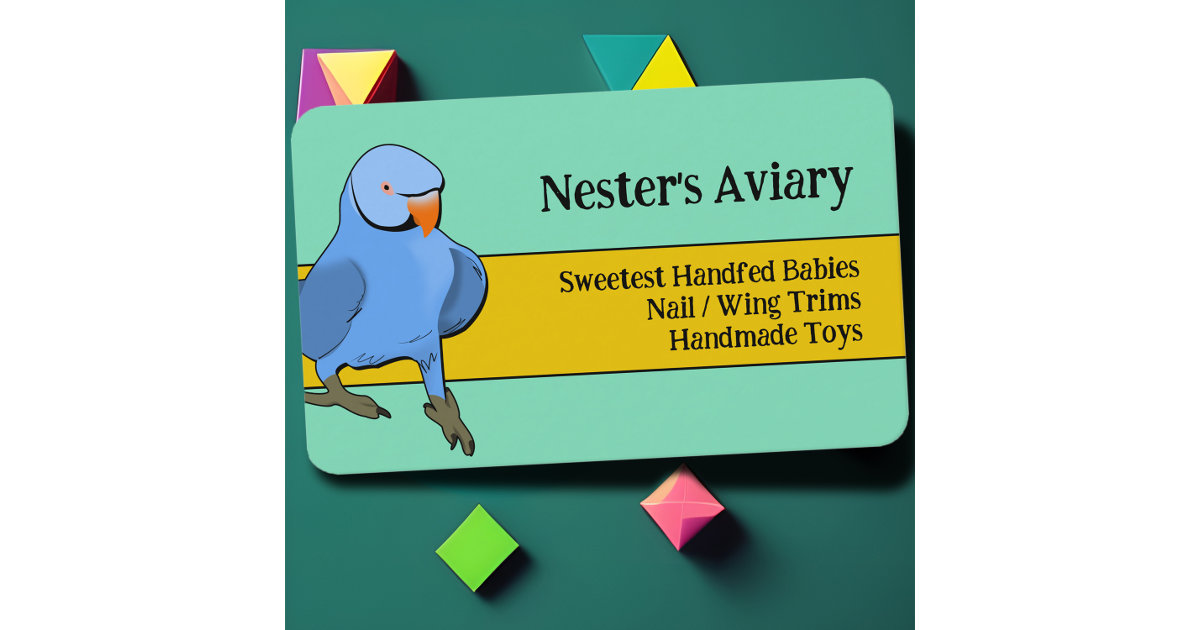The image features a graphic for a company named “Nestor’s Aviary.” The primary background is a dark green, adorned with various geometric shapes: a light green diamond on the bottom left, a pink diamond in the middle bottom, a teal triangle at the top middle, a yellow triangle next to it, and a 3D yellow triangle on the top left with a purple shape behind it.

At the center of this background is a business card with a light greenish-blue hue and rounded edges. On the left side of the card, there is an artwork of a blue bird with an orange beak, orange and black eyes, and brown feet. The card prominently displays the text "Nestor's Aviary" in dark green at the top. Below, a yellow band spans the middle of the card, with the offerings of the aviary listed in dark green: “Sweetest Hand-Fed Babies, Nail/Wing Trims, Handmade Toys.”